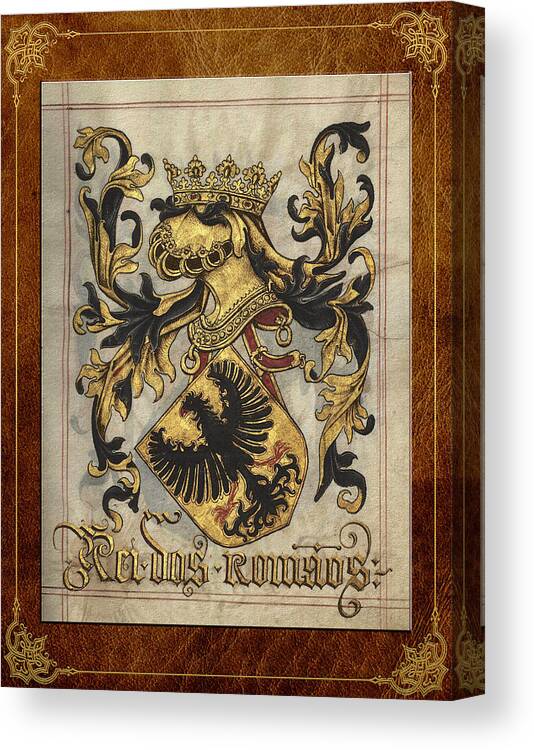This image features a sophisticated piece of artwork displayed on a canvas with a brown, marbled background intended to mimic aged leather. The canvas has a wraparound design and is framed by a thin, ornate gold border with intricate, crown-like swirly patterns at each corner. 

Central to the piece is a white section that houses a strikingly detailed heraldic design. At the top, there is a regal crown resting atop a knight's helmet, symbolizing nobility or royalty. Surrounding the helmet are ornate, flowery designs that add to the decorative elegance of the piece. Below the helmet, a gold shield, oriented sideways, features a black eagle with black projections streaming downwards, enhancing its majestic appearance.

The entire image is rendered in such a way that it gives off a shiny, metallic look, emphasizing its ornamental nature. Beneath the heraldic imagery, there is a gold-colored, scripted text that appears to read something akin to "R-E-I-D-O-S Romanos" or "R-O-M-A-O-S," though the exact wording is difficult to discern due to the artistic script. The overall effect is one of classical elegance, combining modern techniques with a historical aesthetic.